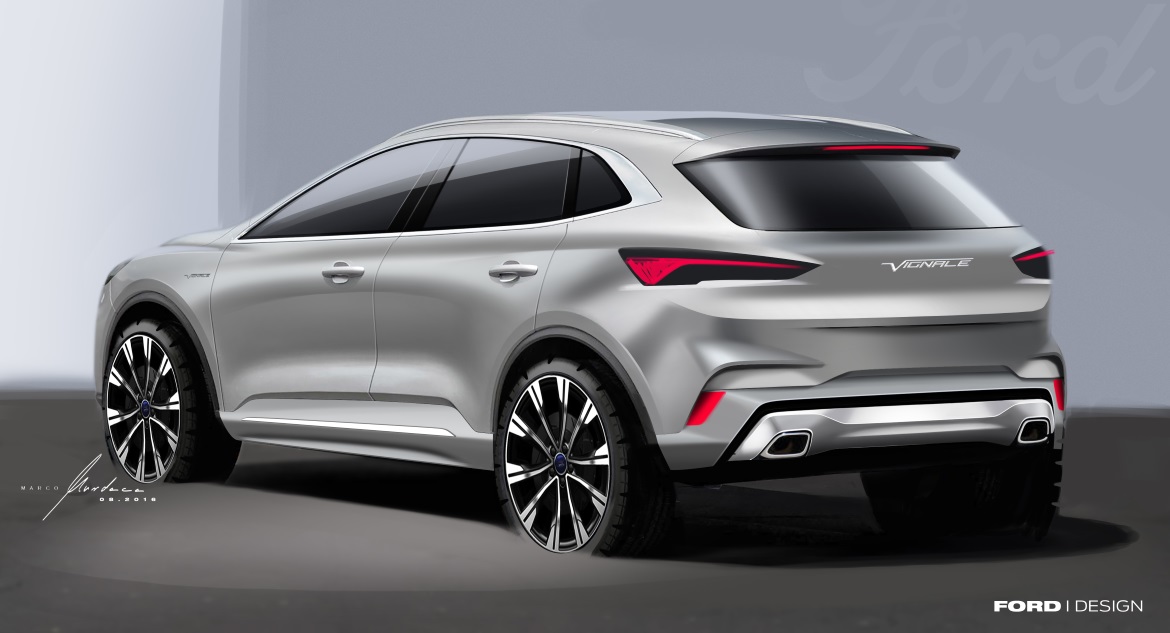The image depicts a detailed rendering of a new car design by Ford, likely intended as a preview. The background consists of varied shades of gray, with the left side appearing whiter and transitioning to a lighter gray towards the center and right. The foreground features a dark gray floor. Prominently centered, the car, identified as a Ford Viennale, is angled about 45 degrees counterclockwise, giving a comprehensive view of its back and partial side. The car is a sleek, lower-profile vehicle, somewhat like a station wagon but lower than an SUV, characterized by tinted black windows and distinctive red taillights. Notable details include a small, cursive signature near the bottom left, possibly by the front wheel on the driver's side, although it is difficult to discern. The car is finished in a sophisticated gray or silver color, accentuating its clean and contemporary design. The branding "Ford" appears in bold white letters in the lower right corner with "design" in thinner letters next to it, while the iconic Ford logo is subtly displayed in cursive at the upper right corner of the image.